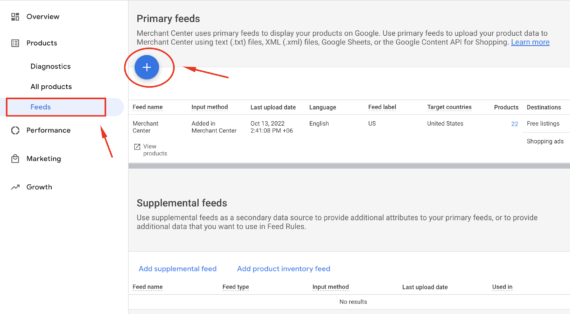The screenshot or recording captures an interface with a highlighted section titled "Feeds" in blue, while the other sections—Overview, Products, Diagnostics, All Products, Feeds, Performance, Marketing, and Growth—are in gray. Under "Primary Feeds," it explains that the Merchant Center utilizes primary feeds to display products on Google. Users can upload product data through various methods, including text (.txt) files, XML (.xml) files, Google Sheets, or the Google Content API for Shopping. A "Learn More" hyperlink is displayed in blue. A blue circle with a white plus sign prompts user actions, while detailed headings such as Feed Name, Input Method, Last Upload Date, Language, Feed Label, Target Countries, Products, and Destinations organize the feed information.